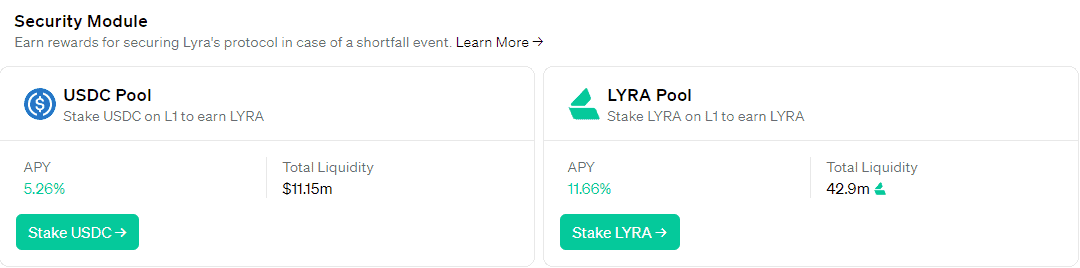The image features a clean, solid white background with text and graphical elements providing information about staking rewards in the Lyra protocol. 

In the upper left corner, bold black text reads "Security Module." Below this, in light gray text, it states: "Earn rewards for securing Lyra's protocol in case of a shortfall event. Learn more," followed by an arrow pointing to the right.

Directly below this information, a light gray box presents details about the USDC Pool. To the left within this box is a blue circle containing a white dollar sign. The accompanying text reads: "Stake USDC on L1 to earn Lyra." Beneath this, in smaller font, the annual percentage yield (APY) is displayed, with "526%" highlighted in green text. Additional details list the total liquidity as "$11.15 million."

Adjacent to this, on the right, another light gray-lined box provides information about the Lyra Pool. The text here indicates: "Stake Lyra on L1 to earn Lyra." Below this, in gray text, it again mentions the APY, showing "11.66%" in green text.

The overall layout is well-organized, offering clear and concise information about staking options and potential rewards within the Lyra protocol.